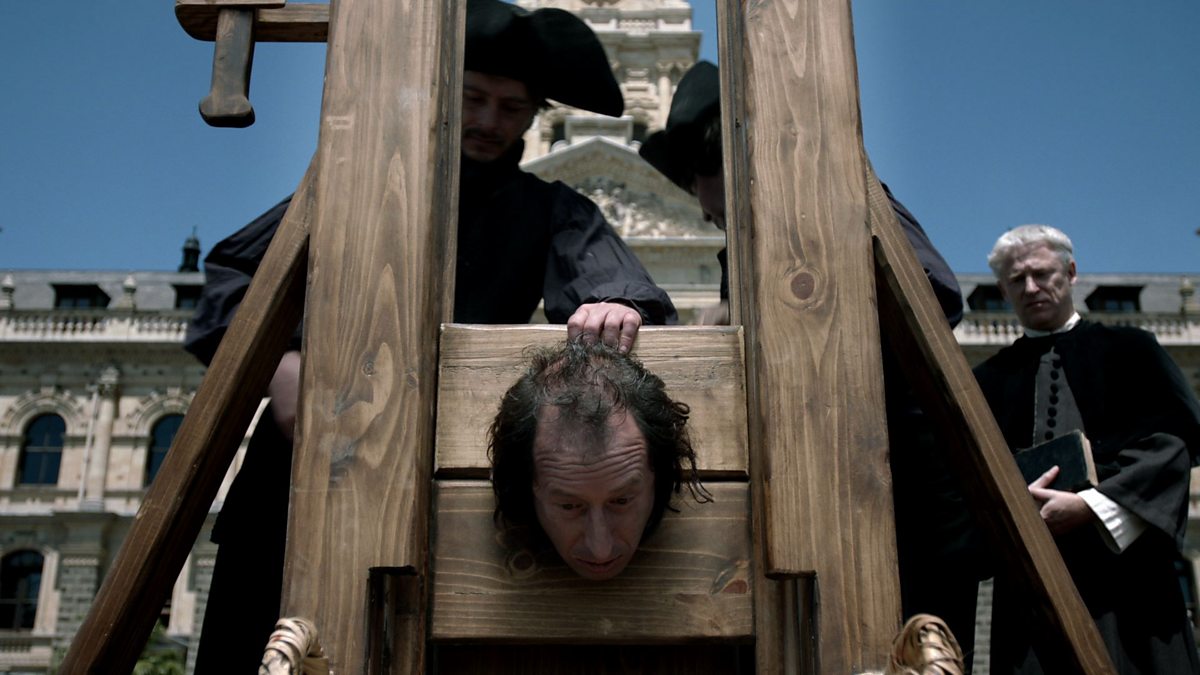This outdoor daylight photograph captures a historical reenactment of an execution scene centered around a guillotine. The focus is on a man with fair skin and dark, somewhat balding hair, whose head is nervously protruding through the wooden boards of the guillotine. He appears bewildered with wide-open eyes. The wooden structure of the guillotine, dark brown and grainy, rises upright with two large beams supporting it.

Behind the man in the guillotine, another figure dressed in colonial-era attire, including a black robe and a large three-cornered hat, is seen placing or securing the victim's head. Adjacent to him stands a priestly figure, an older man with white hair styled in a bowl cut, wearing a black robe and white shirt, holding what appears to be a black Bible.

The setting is further contextualized by the backdrop of a grand, off-white stone building featuring dark arched windows and columns, suggestive of colonial architecture. The clear blue sky further enhances the historical ambiance of the scene. The overall impression is that of a captured moment from a video or film, providing a vivid depiction of an old-time execution.